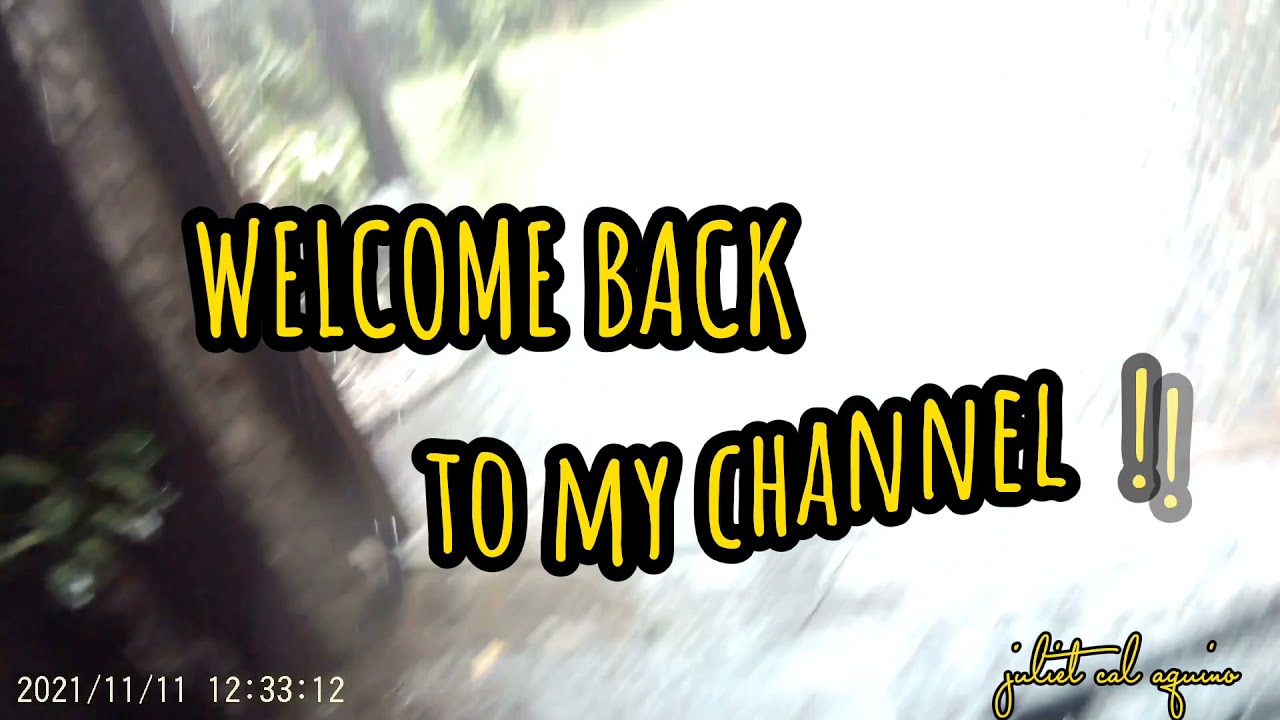This image appears to be a banner-style screenshot, reminiscent of a YouTube channel interface, captured from outdoors in the middle of the day. Central to the image is the text "Welcome back to my channel!!" in yellow lettering. A blurred and bright ball of light is positioned centrally behind the text, obscuring much of the background. Raindrops are visible around the light, suggesting it is raining. Surrounding this bright spot, the background scenery includes part of a building with visible plants, sunlight, and possibly some palm trees to the left. There is a thin, dry, and brick-style rectangle visible on the left, hinting at a corridor, doorway, or garage. The timestamp "2021/11/11 12:33:12" is located in the bottom left corner, while a gold cursive signature, possibly reading "Juliet Cal Aquino," appears in the bottom right. The text and weather elements combine to create a unique and engaging banner design against a varied yet somewhat obscured outdoor backdrop.